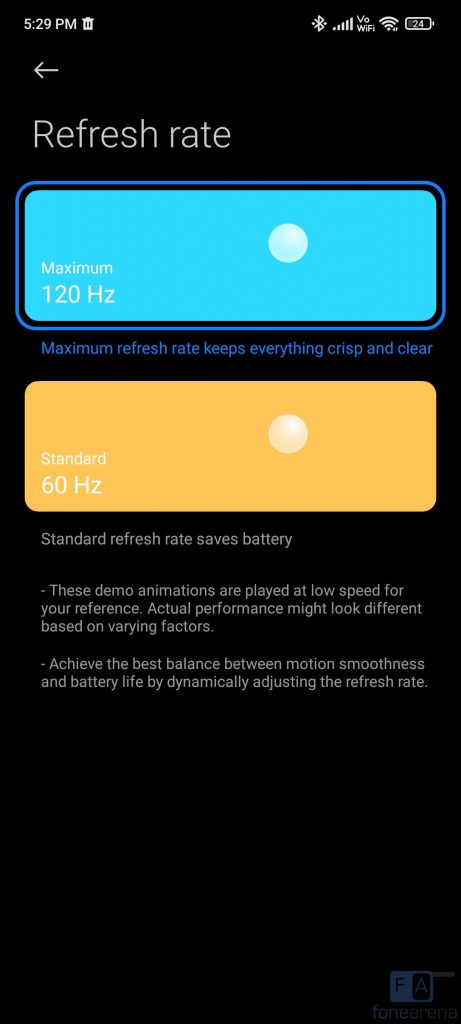The image depicts a mobile app interface with a detailed status bar at the top. In the upper left corner, the time is displayed as 5:29 PM, accompanied by a trashcan icon. On the right side of the status bar, several icons are visible: a Bluetooth icon, a five-bar signal strength icon, text indicating "VO Wi-Fi" alongside a full Wi-Fi icon, and a battery icon showing 24% charge.

Just below the status bar, a white arrow pointing left serves as a back button, and next to it, "Refresh Rate" is written in white font. 

Central to the interface is a prominent button in bright sky blue, featuring a black and blue border. This button reads "Maximum 120 Hertz" and includes a description: "Maximum refresh rate keeps everything crisp and clear."

Below the blue button, an orange rectangle without a border states "Standard 60 Hertz," accompanied by the text: "Standard refresh rate saves battery."

Further down, a text note explains: "This demo animations are played at low speed for your reference. Actual performance might look different based on varying factors. Achieve the best balance between motion smoothness and battery life by dynamically adjusting refresh rate."

In the bottom corner of the image, the word "FONEARENA" (stylized as "F-O-N-E-A-R-E-N-A") is visible, all set against a black background.